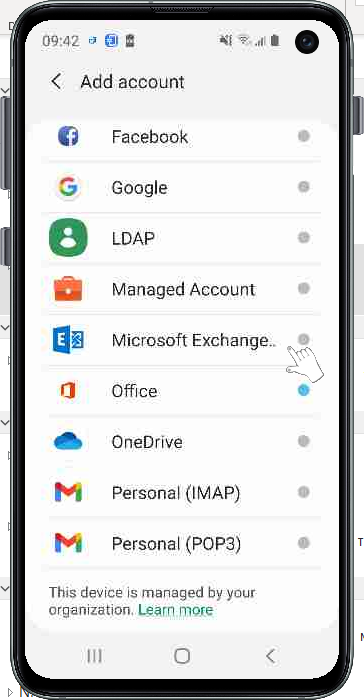This image appears to be a detailed simulation of a cell phone's screen, resembling an informational graphic or a settings menu interface. The simulated screen displays a smartphone with various elements and icons:

1. **Top Bar:** 
   - Time: 9:42
   - Blue icons indicating battery level and Wi-Fi status.

2. **Profile Section:**
   - A black circle serving as a profile picture placeholder.
   
3. **Background & Font:**
   - Background: Predominantly white and gray.
   - Text: Black font used for labels and descriptions.

4. **Settings Menu (App List):**
   - **Facebook:** Blue and white Facebook logo.
   - **Google:** Multi-colored 'G' within a white circle.
   - **LDAP:** Green square with a white person icon.
   - **Managed Account:** Orange briefcase icon.
   - **Microsoft Exchange:** White cartoon hand icon pointed towards it.
   - **Office:** Red-orange icon.
   - **OneDrive:** Blue and light blue cloud icon.
   - **Personal (IMAP):** Gmail icon with shades of blue, red, yellow, and green.
   - **Personal (POP3):** Repeated Gmail icon with a similar color scheme.

5. **Footer:**
   - Message: "This device is managed by your organization" in gray text.
   - Learn More button in green.
   - Additional symbols: Three lines, a square box, and an arrow.

6. **Overall Layout:**
   - The fake cell phone image is black with a simulated layered effect showing the gray background with white and black text.

This realistic depiction highlights an organized and structured settings menu with identifiable icons and labels, effectively mimicking a real smartphone interface.